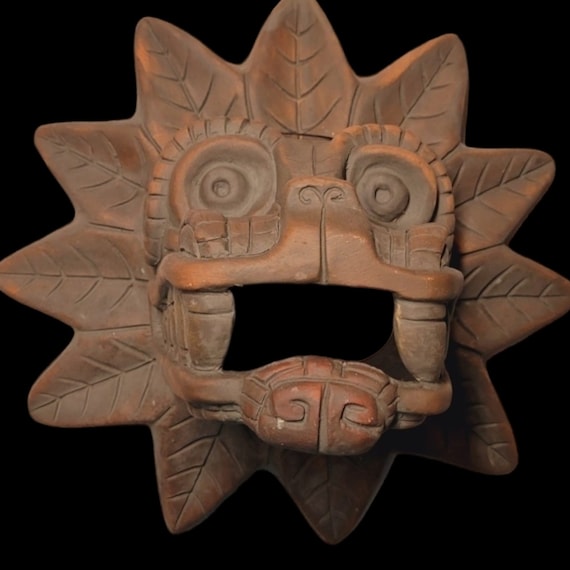In this striking photograph, a close-up of a pre-Columbian terracotta clay artifact is meticulously presented against a stark black background, accentuating its antiquated beauty. The sophisticated lighting employed in the shot casts a radiant glow on the orange terracotta, bringing the textures and intricate details of the piece to life. The artifact features a vividly detailed full-frontal visage of what appears to be a monstrous or reptilian face, mouth agape to reveal a shadowy interior. Surrounding the face is a fan-like arrangement reminiscent of a starburst, adding to its dramatic visual impact. Although the exact scale of the artifact is not specified, the craftsmanship is undeniably captivating, blending detailed design with a primitive aesthetic. This clay piece is a palpable echo of pre-Columbian artistry, captivating in both its historical significance and its picturesque presentation.